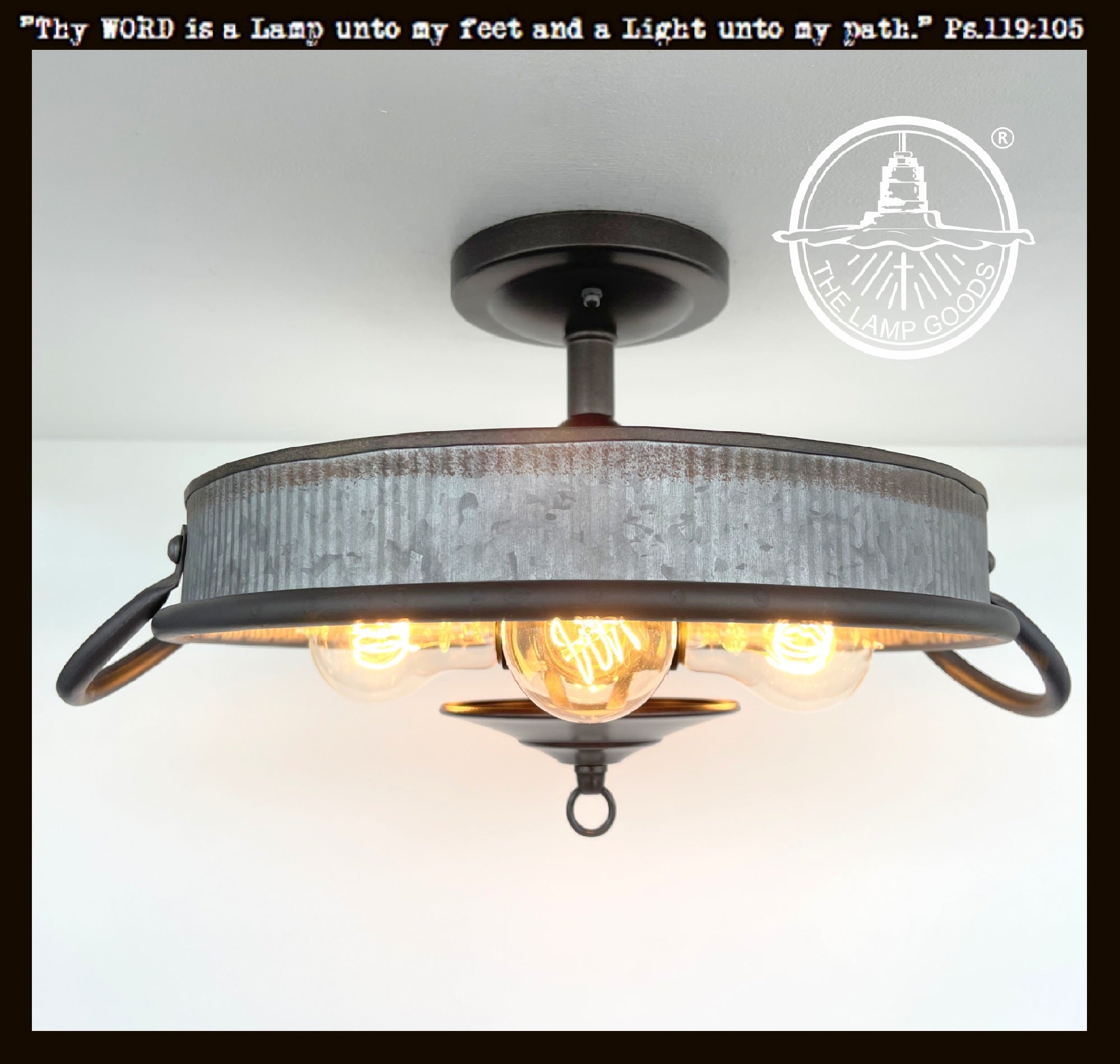The photograph features a distinctive ceiling lamp, ingeniously crafted from a repurposed silver cooking pot or thin pan, with two metal handles protruding from both sides. The lamp itself is suspended from a black ceiling mount against a white ceiling and wall. Three exposed light bulbs glow warmly from within the cylindrical pot, showcasing their yellow light. Below the pot, a typical round, funnel-shaped cover commonly found on metal ceiling lamps is absent, leaving the bulbs fully visible. A white logo reading "The Lamp Goods" with an icon of a lamp is positioned in the upper right corner. Above the lamp, a black banner displays the text in white, "Thy word is a lamp unto my feet and a light unto my path," attributed to Psalms 119:105.